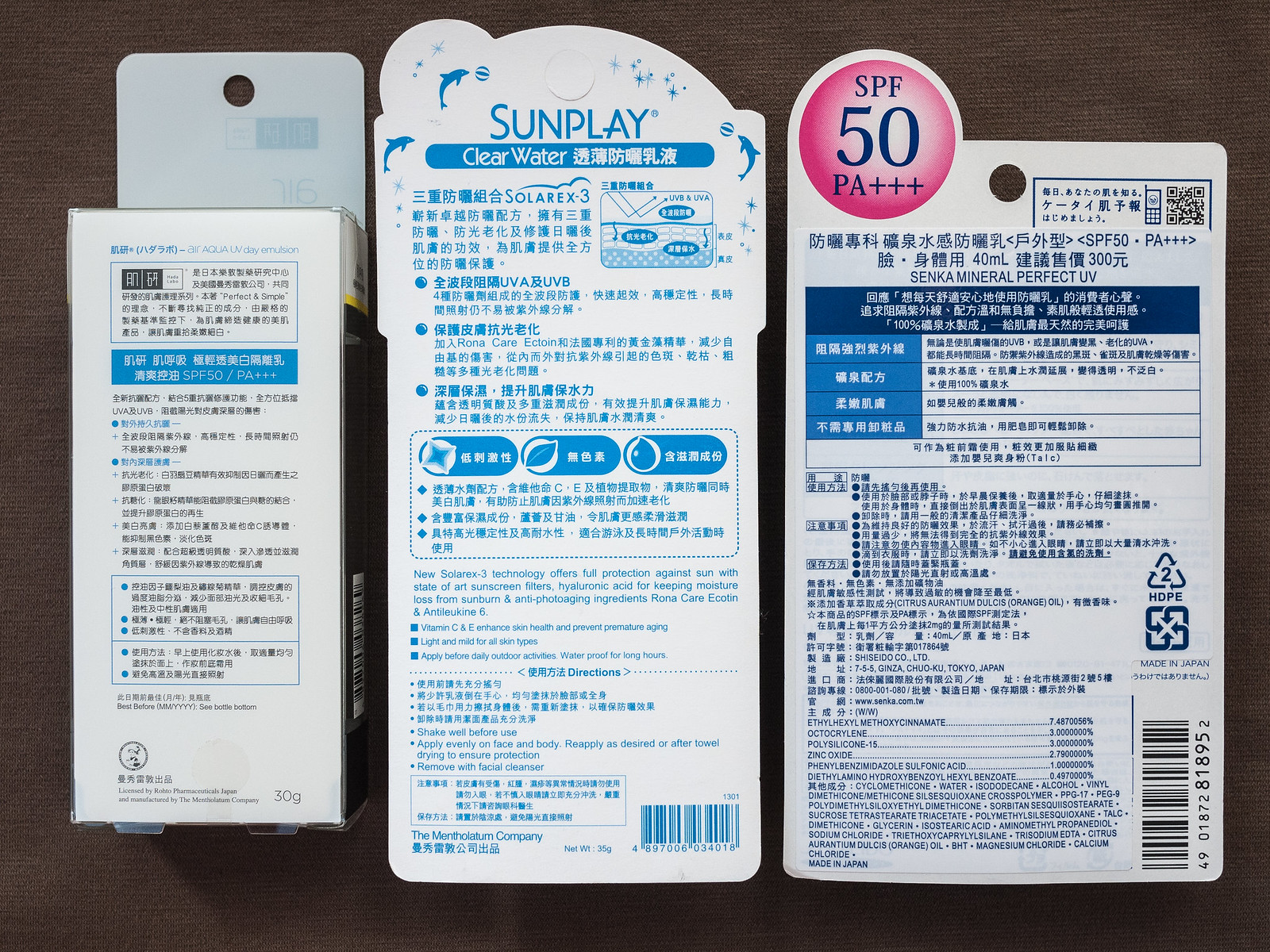The image is a color photograph showcasing three different packages of consumer products, likely sunscreen, with cardboard packaging. The majority of the writing on these packages is in what appears to be traditional Japanese symbols, although the text is slightly blurred. Visible on the middle and right packages are barcodes: the middle package features a navy dark blue barcode, while the package to the right has one in black ink.

The rightmost package includes a notable pink circle in the top-left corner. Inside the circle, the text reads "SPF 50 PA+++" in navy blue, indicating a high sun protection factor. The middle package prominently displays the word "SUNPLAY" in capital letters at the top in English, along with the words "CLEAR WATER" in white below it. This package also features illustrated dolphins, shadow-filled in an arc, appearing to jump out of the water in the top left area of the package. 

Collectively, these packages likely constitute a set of various sun protection products. The middle package, "Sunplay Clear Water," and the third one with SPF details suggest sunscreen products suitable for different consumer needs.